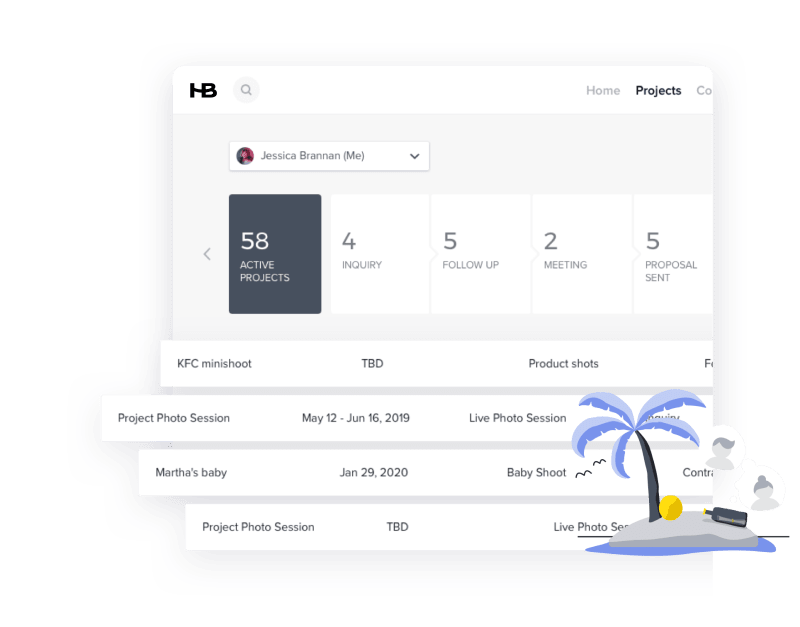The image is a detailed illustration of a photographer's project management dashboard on a website. At the top section, set against a white background, the left corner features the initials "HB" accompanied by a search icon. On the right side, navigation options "Home" and "Projects" are displayed, with "Projects" highlighted. At the top left, a profile scroll bar shows the name "Jessica Brannon, me."

Below the navigation bar, there's a section of slider boxes. The first slider box, highlighted in grey, indicates "58 active projects." Following categories are listed as "4 inquiry," "5 follow up," "2 meeting," and "5 proposal sent." Beneath this section, four horizontal white bars are offset, each detailing different projects:
1. "KFC Mini Shoot, TBT product shots."
2. "Project Photo Session, May 12 to June 16, 2019 live photo session."
3. "Martha's Baby, January 29, 2020 baby shoot."
4. "Project Photo Session, TBD live photo session."

At the lower right-hand corner, an illustration depicts a blue palm tree on a grey rock, accompanied by a black bottle and a yellow circular object. The rock appears to be situated on a blue lake, with two circular empty profile icons floating above the bottle. The entire setup effectively organizes and displays the photographer's various shoots, their dates, and specific details about each session.